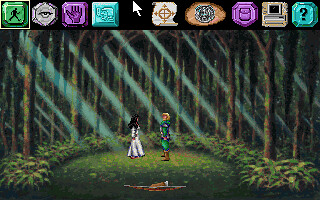A detailed screen capture of a vintage video game, specifically reminiscent of early portable or handheld gaming devices. The image's low-resolution pixelation highlights its simplistic and nostalgic design. At the top, vintage-styled icons are visible, including profiles of human faces, eyes, hands, helmets, a compass, medallions, a pocket, a retro computer desktop layout, and a question mark, evoking the era's limited graphical capabilities and imaginative interface elements.

The main scene features a woodland background with lush trees and ferns, enclosing a semi-circular arena. In the center, two characters face each other, seemingly preparing for battle. One character is depicted in white, while the other is adorned in armor, enhancing the game's medieval or fantasy theme. The overall ambiance is distinctly vintage, pointing to a simpler, earlier stage in video game history, far removed from the current high-tech standards.